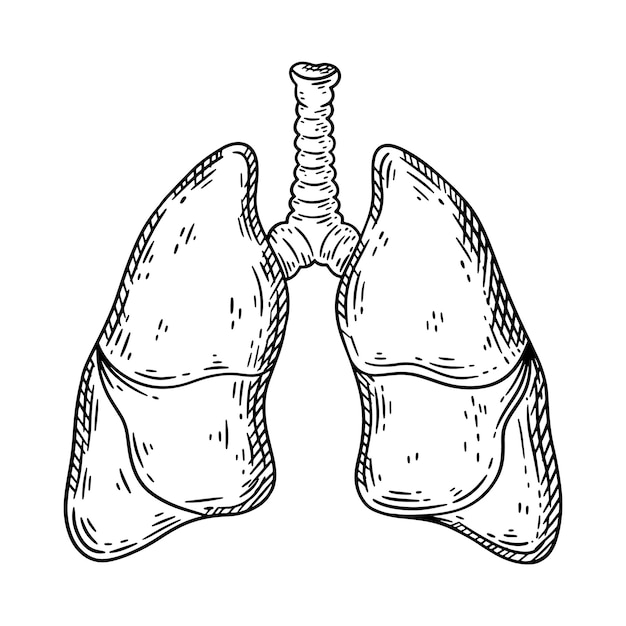The image is a detailed black and white line drawing of a pair of human lungs connected to the trachea. The drawing features the ribbed structure of the trachea, which branches into two large, multi-chambered lungs, each appearing to be divided into three segments. The style of the illustration is cartoony yet serious, utilizing cross-hatching for shading, especially along the edges. The background is completely white, and the image is devoid of any text, labels, or additional structures, giving it a simplistic and uncluttered appearance. The lungs are outlined in black, and the overall composition suggests it could be used in a medical book or encyclopedia.